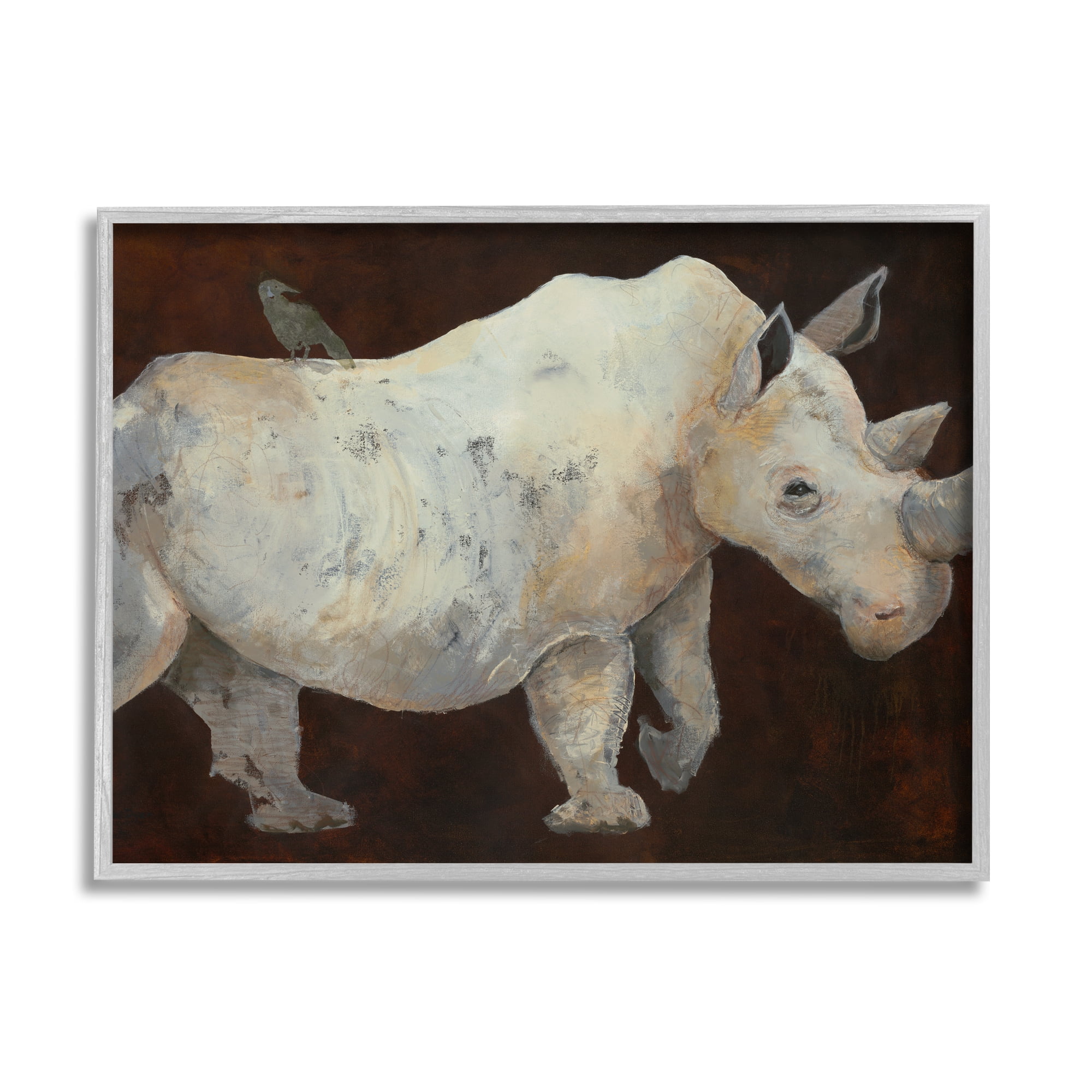In this intricate art piece, a rhinoceros, likely a white rhino due to its predominantly white and gray coloring with touches of brown and tan, is depicted moving from left to right. Its head faces right, and its left foreleg is raised mid-step. The background is dark brownish, textured with splotches of black and hints of muted reds, which give it depth and complexity. The rhino's ears are perked forward, and a small black bird perches on its back. The rhino's body is detailed, with a significant belly that sags slightly, showing a lifelike realism. Notably, its right eye is visible and seems to gaze at the viewer, adding a sense of presence. The rear right leg and tail are out of frame. This painting is enclosed in a thin white frame that enhances the piece without distraction. The overall texture of the rhino almost gives it a plastic-like illusion amidst the richly detailed and expressive background.